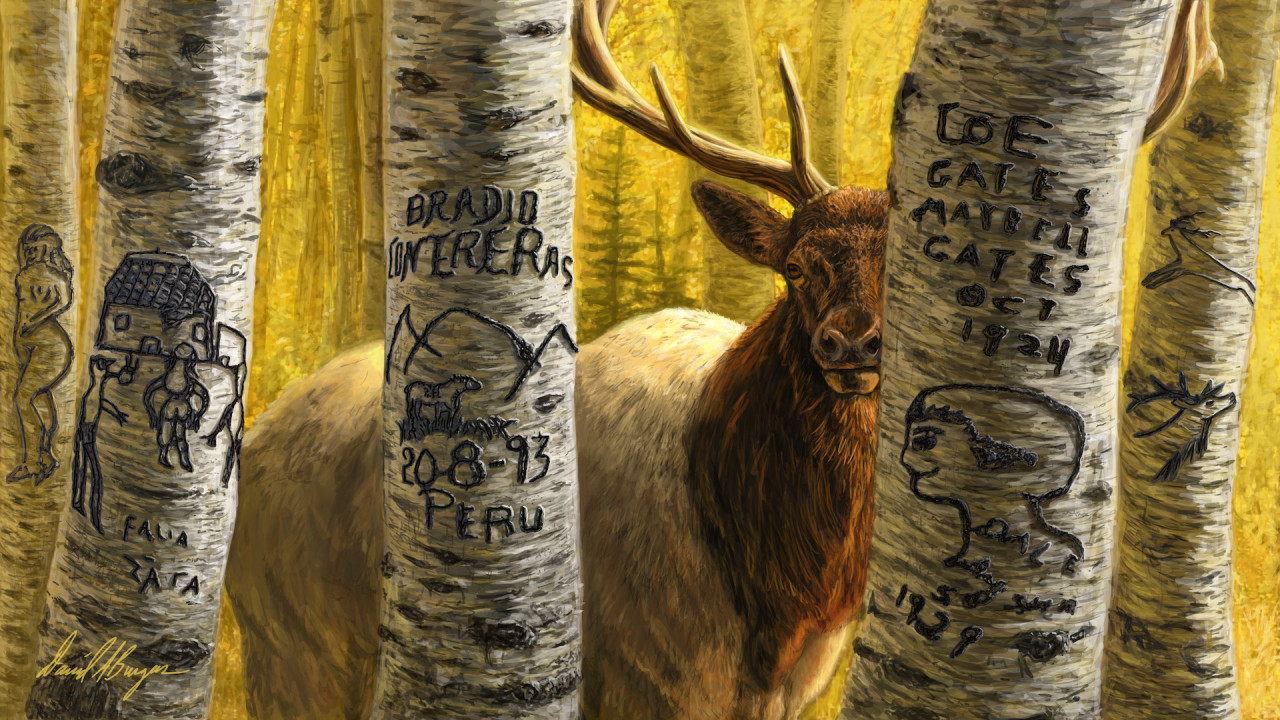The painting depicts a serene forest scene with several beech-like trees. Carved into their trunks are various images and writings, each telling its own story. Among the carvings are a signature from "Mattrell Gates, Oct. 1924," depictions of a house with people walking towards it, a jumping reindeer, reindeer heads, a naked woman, and the phrase "C-O-E-G-A-T-E-S." Prominently, a majestic buck deer with large antlers stands amidst the trees, gazing directly at the viewer. The buck has a brown head and neck, transitioning to a lighter brown body. The antlers, equally impressive, are a beige-brown color, with the right set fully visible and the left partially obscured by the trees. A golden signature is located in the bottom left corner of the painting, adding a final touch of authenticity to the intricate artwork.